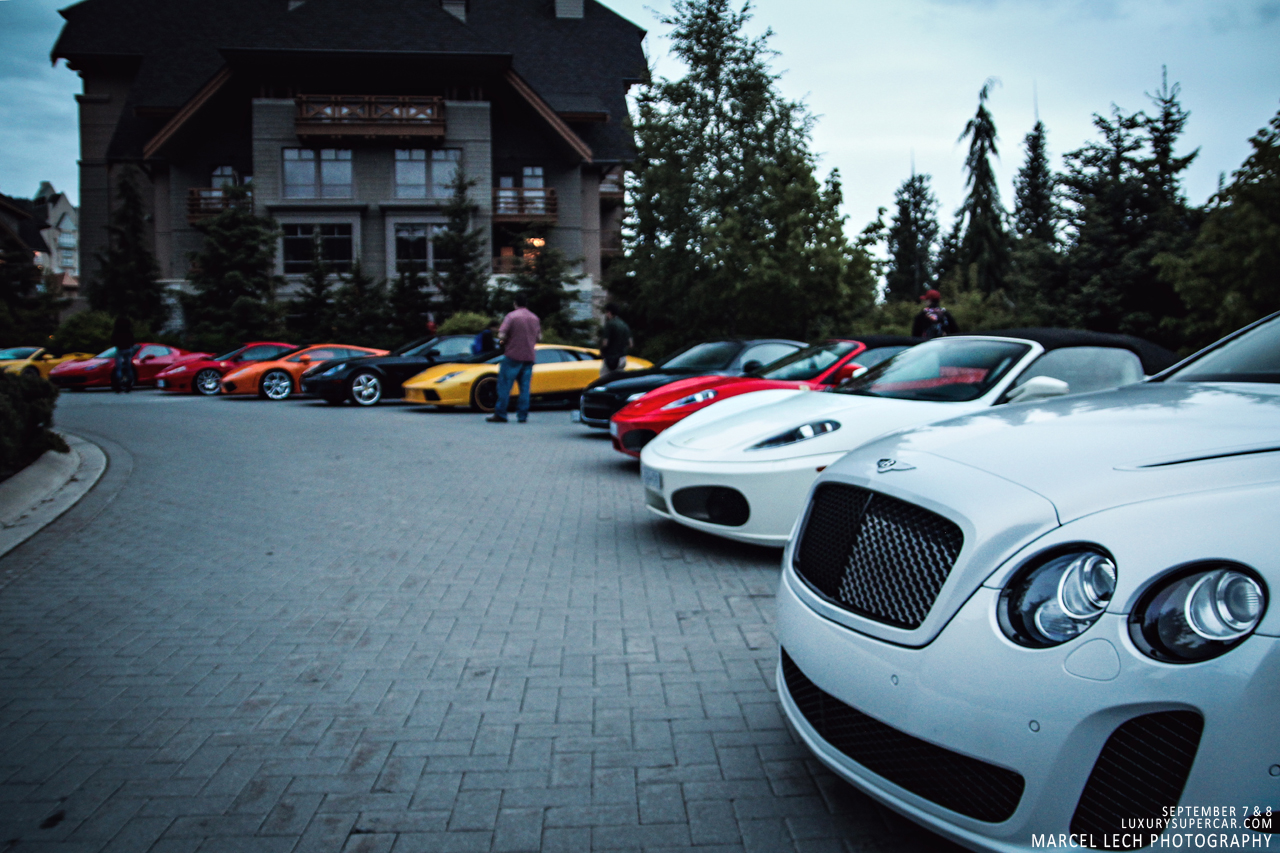A luxurious car show unfolds on the expansive brick driveway of an imposing lodge-like mansion that stands tall in the background with its dark brown facade and grand windows. The driveway, paved with cobblestone and forming a circular pattern, showcases an impressive lineup of exotic sports cars. At the forefront, a pristine white sports car is followed by a sleek red convertible and a striking yellow sports car, around which two admirers stand. The collection features a total of around ten high-end vehicles, including several red, black, and yellow models, all meticulously parked with their front ends facing outward in a semi-circle. The presence of evergreen trees adds a touch of greenery to this otherwise opulent scene, under a bluish-gray sky hinting at an overcast day. Captured by Marcel Lech Photography and noted on luxurysupercar.com, the scene is set on September 7th and 8th of an unspecified year, perfectly framing the allure and sophistication of these magnificent machines.